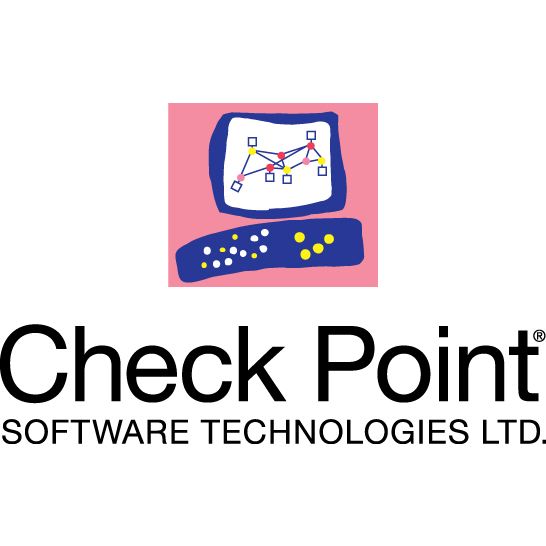The image is a detailed business logo for Checkpoint Software Technologies LTD. The logo is set against a white background. The top half features a pink square containing an abstract, animated depiction of a computer. The computer has a blue border around the screen and a keyboard or remote control below it. The screen is filled with interconnected elements, including yellow, red, and pink dots, blue lines, and white squares with blue borders. The keyboard, represented in blue, features various illuminated white and yellow dots. Below the pink square, the company's name is displayed in bold black text: "CHECKPOINT" in large letters, followed by "SOFTWARE TECHNOLOGIES LTD" in smaller print.